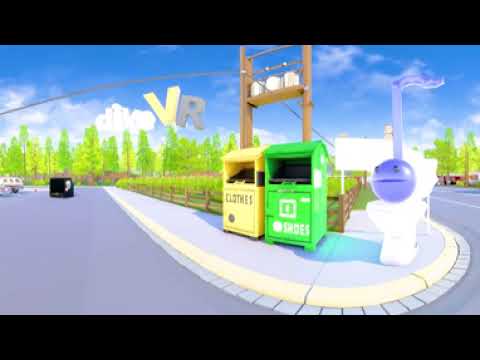The image depicts a detailed 3D digital scene of an outdoor city street environment, resembling a painting with a cement walkway curving out towards the viewer, surrounded by grey bricks. To the right, there is a peculiar white toilet with a blue ball on top that has a face with eyes and a mouth, resembling a musical note with a stem rising upwards. In the center, there are two prominent donation bins: the green one indicates "shoes," while the yellow one is labeled "clothes" for recycling purposes. Beyond the bins lies a fence adorned with some greenery and shrubbery, adding to the serene background. Behind the bins, two poles can be seen mounting a structure that seems to have three containers. In the far distance, buildings and a smokestack emitting smoke are visible, suggesting an urban setting. The sky above is blue with scattered clouds and features yellow letters "VR," with white letters spelling "DIVE" or "DIXE" in front of them. Additionally, a vehicle, described as square and black, is positioned on the left side of the scene.